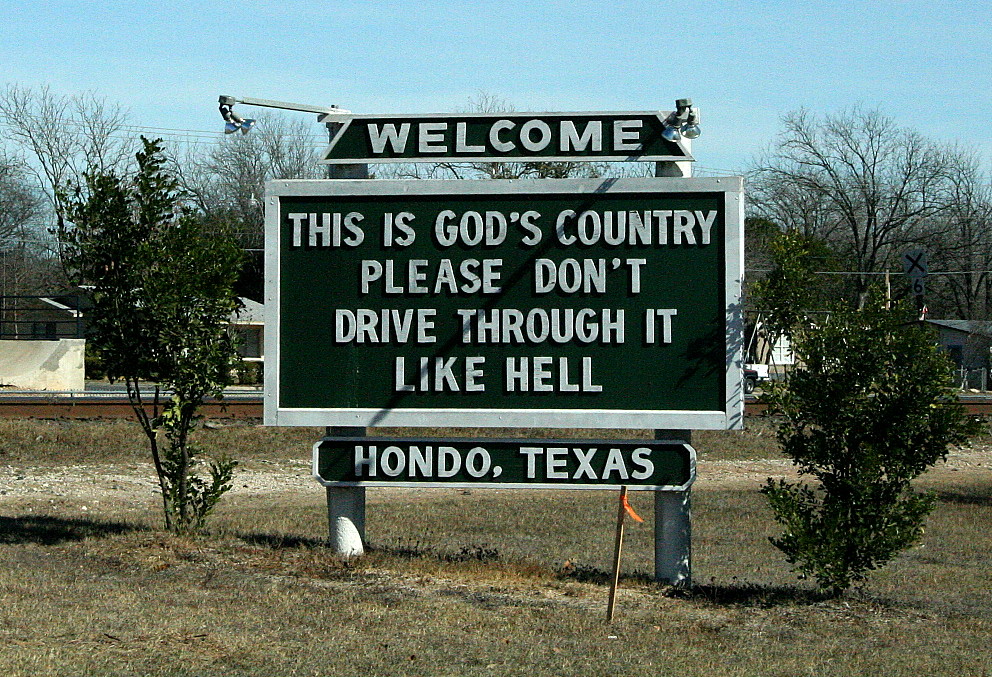The image captures a prominent outdoor sign situated in a field with dry, brown grass. The backdrop features a clear, blue daytime sky and a stand of smaller trees or shrubs flanking the sign. The sizeable sign, bordered in white, prominently displays the word "Welcome" at the top. Below it, in bold white letters against a black background, the sign reads, "This is God's country, please don't drive through it like hell." At the bottom, the sign designates its location with "Hondo, Texas." A noticeable feature in the foreground is a wooden stick topped with an orange flag, planted firmly in the ground. Additionally, there are lights mounted on the top and side of the sign, enhancing its visibility.